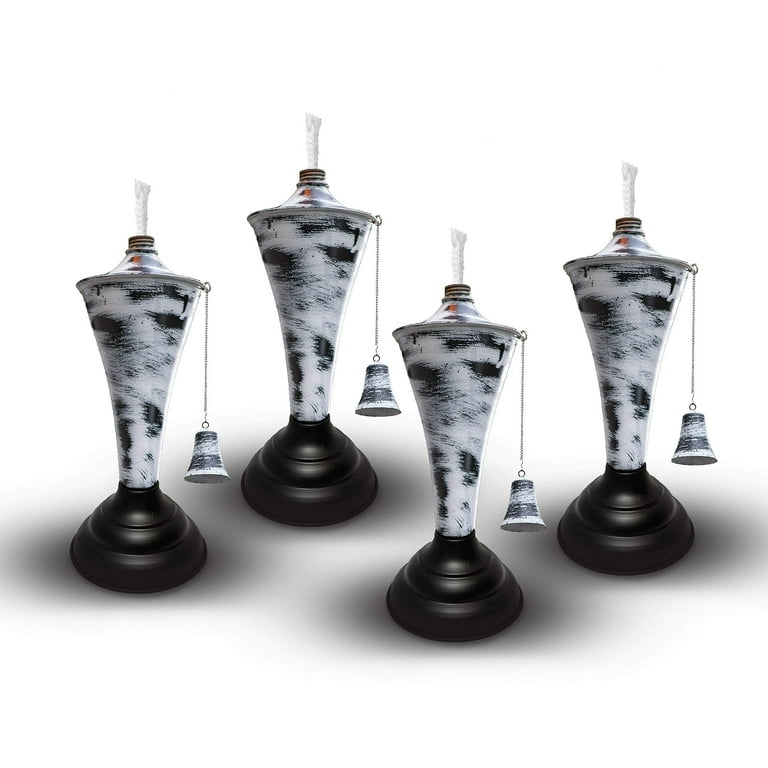This image showcases four identical oil torches, each designed to be mounted on a dowel, often used for outdoor gatherings. These elegant torches, likely created through AI rendering, feature a black and white, tornado-like design that transitions into a brown base. Each torch is topped with a thick, white cotton wick, which extends about an inch above the oil reservoir. To extinguish the flame, a small chain hanging from each torch holds a cap that can be placed over the wick, cutting off its oxygen supply. These torches are likely filled with citronella or another type of oil, making them ideal for lighting up a yard during a party or for emergency use during power outages.